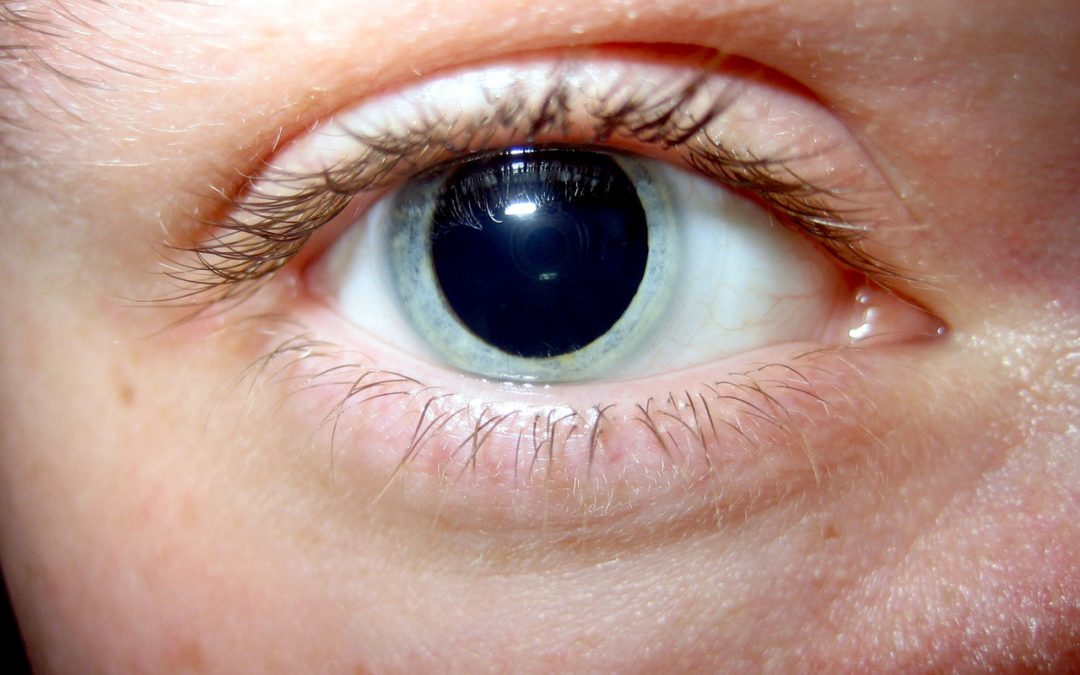This photograph is an extreme close-up of a Caucasian person's eye, focusing intensely on the eye itself which occupies most of the frame. The light-skinned face reveals minimal features: just a few hairs from the eyebrow in the top left corner, a tiny portion of the nose, and a hint of the cheek below the eye. The pupil is strikingly dilated, occupying almost 90% of the visible eye area, with a thin strip of light blue, almost white, iris encircling it. The iris appears unnaturally light and thin, suggesting the possibility of the person wearing a contact lens. The sclera (white part of the eye) shows faint red lines, hinting at slight bloodshot areas. The black eyelashes curve naturally above the eye, reflecting subtly in the pupil. The eye is normally open, not exaggeratedly so, framing a mesmerizing gaze that captivates the viewer with its peculiar intensity.